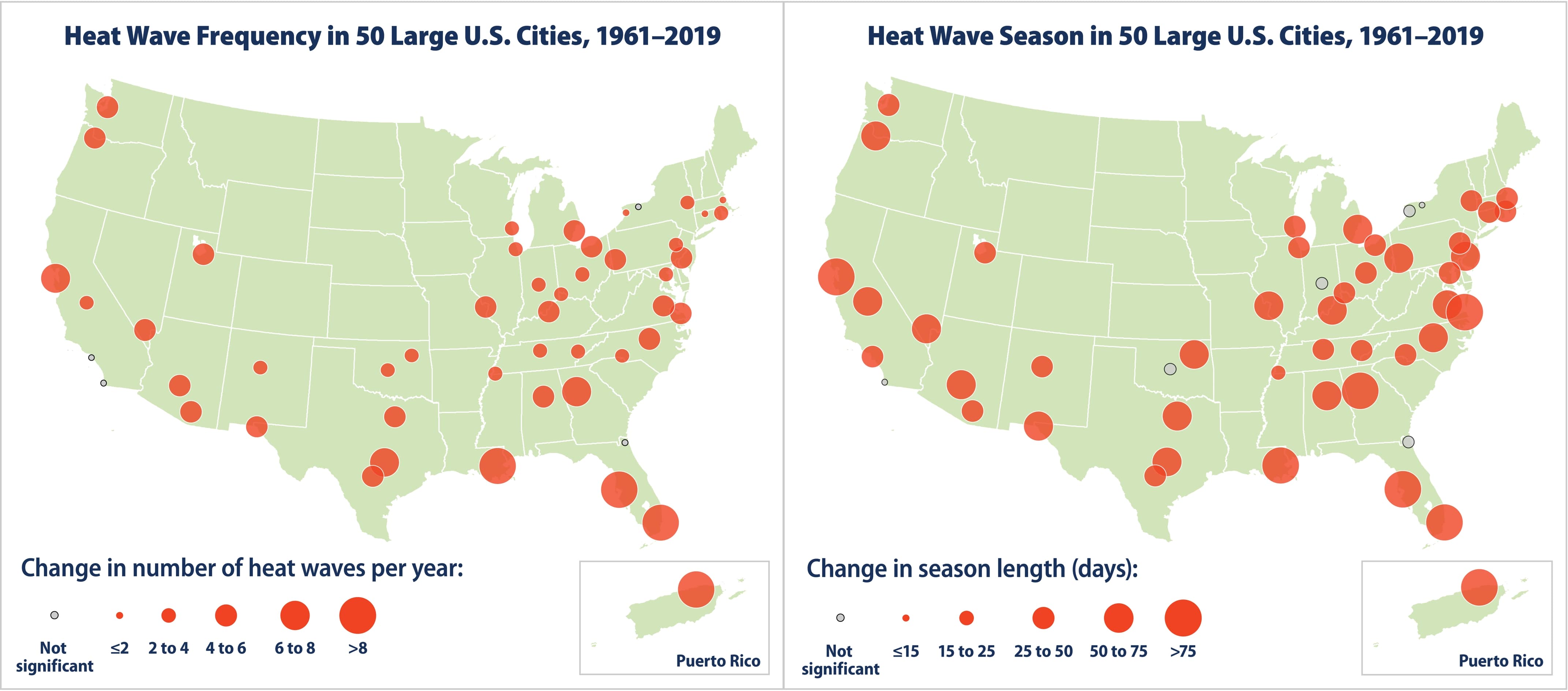The image consists of two side-by-side maps of the United States, both shaded in a very pale green, set against a white background. Each map focuses on different aspects of heatwaves in 50 large U.S. cities from 1961 to 2019. The map on the left, titled "Heat Wave Frequency in 50 Large U.S. Cities 1961-2019," features red circles that vary in size to represent the change in the number of heat waves per year across the cities. The larger the circle, the greater the change in heat wave frequency. The map on the right, titled "Heat Wave Season in 50 Large U.S. Cities 1961-2019," similarly uses variably sized red circles to denote changes in the length of the heat wave season, measured in days. At the bottom of each map, there is a key that explains the significance of the circle sizes. Both maps aim to convey the impact of climate change on heatwaves across various U.S. cities, with notable differences in frequency and season length illustrated through the distribution and size of the red circles.